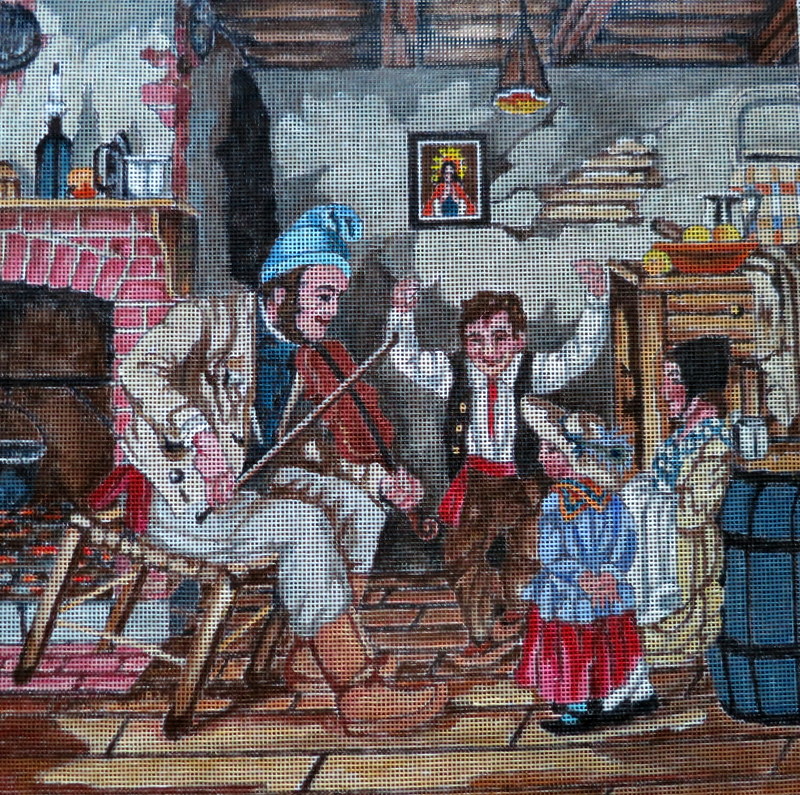The image appears to be a detailed cross-stitched or tapestry scene set within an old, rustic cottage. A bearded man, dressed in a blue hat and a brown suit, is seated on a woven wooden chair, playing a fiddle. He leans forward, and his chair tilts on two legs, adding a sense of movement to the scene. Gathered around him are three children, dressed in attire reminiscent of mini adults—a boy in a white shirt, red tie, black vest, red sash, and brown pants, and two girls: one in a straw hat with a blue feather, a blue shirt, red and orange accents around her neck, a red skirt, and blue socks with black shoes; the other with a black hat, wearing a dress that is blue and white at the top and khaki and brown below, complemented by an apron.

In the backdrop, there is a white wall with peeling plaster revealing brickwork, adding to the historical ambiance. A framed portrait of Jesus hangs on the wall. To the left, a large fireplace features a pot hanging over it and a mantle adorned with various items, including a blue bottle and a candle. On the right side, several shelves or drawers hold a red bowl with fruit and assorted objects. Below the roof, which has a wooden log texture, a wooden chandelier hangs, enhancing the cozy yet worn charm of the cottage. A blue barrel near the children adds to the scene's depth, with what seems to be a coffee cup placed on top. The totality of the image gives the impression of a grainy, textured, handcrafted piece, rich in historical and cultural detail.